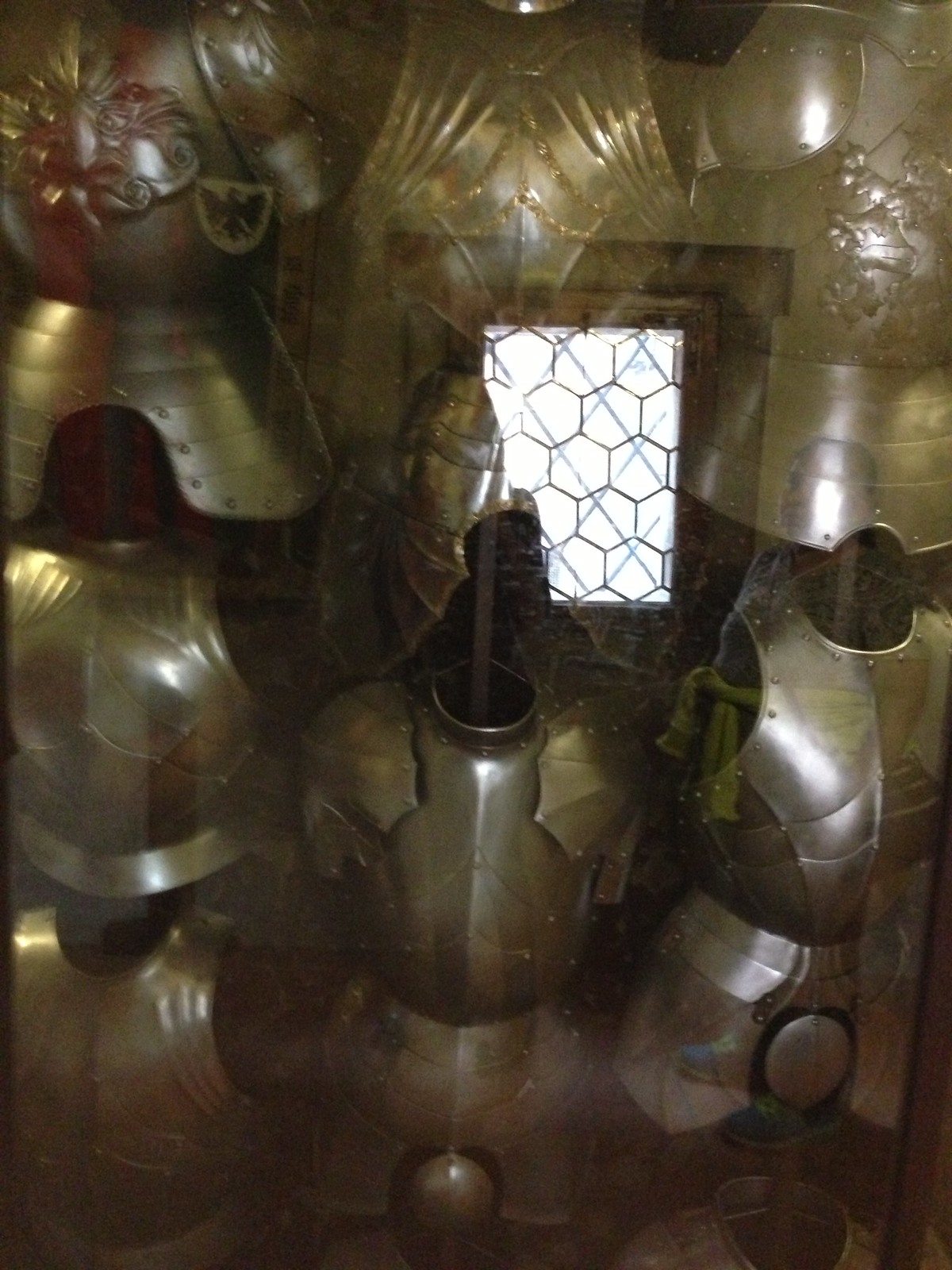This is a surreal, AI-generated color photograph taken indoors, characterized by a surreal and dreamlike quality. Dominating the middle and extending towards the upper left corner, there is a square window framed by a large brown wooden door frame, behind which emanates a bright white light filtered through an almost hexagonal mesh or chicken wire. Surrounding this central feature, the image showcases several pieces of metallic, silver-colored armor positioned vertically, as if mounted on black poles. These armors, which lack headpieces, display various levels of intricacy; the upper sections are prominently detailed with embossing and ornate designs that include floral patterns and a lion motif on the center-right chest piece. The lower chest pieces, by contrast, are much plainer and feature notable round silver circles near the hip area. The entire scene has an ethereal, semi-translucent appearance, giving the impression that the armor is ghostly or superimposed over the backdrop. To the upper left, a subtle reddish tinge enhances the otherworldly ambiance of the photograph.